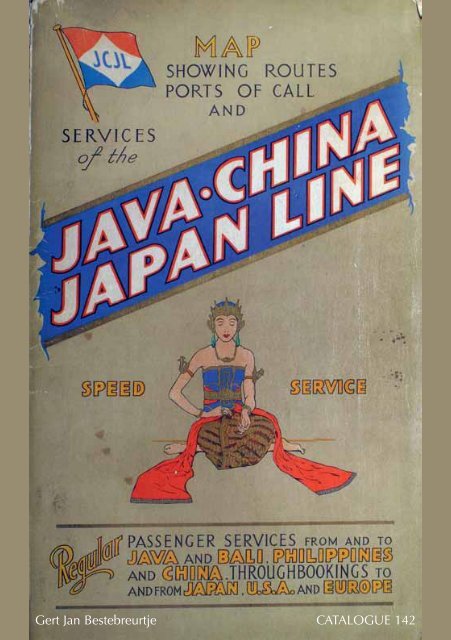This is the front cover of an old and somewhat damaged travel catalog, marked catalog 142. The top of the catalog features the text "Map Showing Routes, Ports of Call," which is highlighted in yellow and sets the stage for the travel-related information within. Below this, a blue banner prominently displays the words "Java China Japan Line," indicating the primary geographic regions served. On the left side, the word "Speed" is written in gold, and on the right, "Service," suggesting the quality of the travel offerings.

Central to the cover is an illustrated woman wearing a blue strapless dress, along with straps on her biceps. She is pulling a red scarf out of a brown bag, adding a touch of elegance and motion to the design. The bottom of the cover lists the detailed services provided, stating "Passenger services from and to Java and Bali, Philippines, and China through bookings to and from Japan, USA, and Europe," emphasizing the extensive travel routes available. Additionally, the name Gert Jan Westenbert appears at the bottom, possibly indicating the creator or an important figure related to the catalog. Overall, this catalog appears to promote a historical connection and comprehensive travel services throughout Asia and beyond.